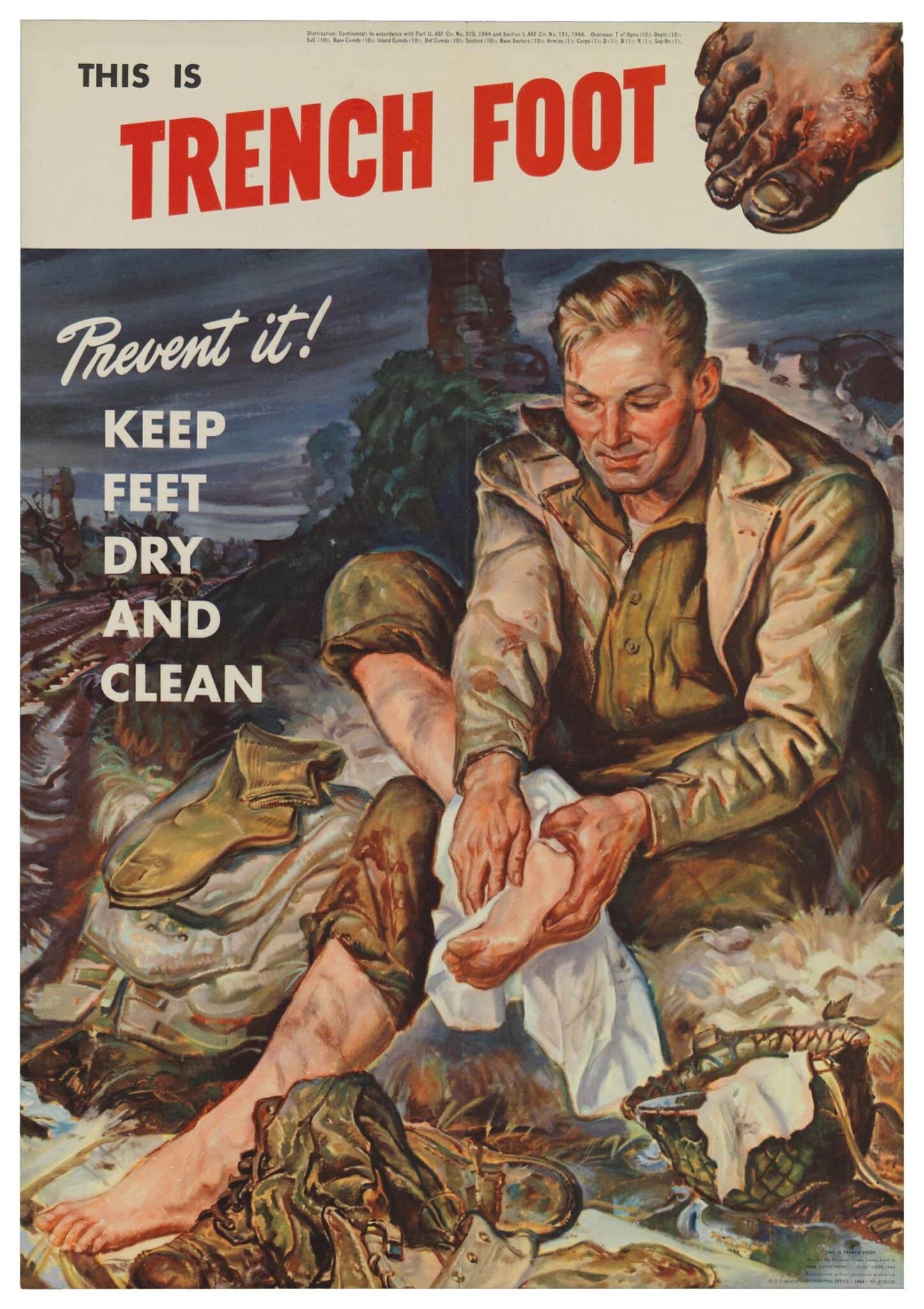The image resembles an old World War I or World War II propaganda poster. At the top of the poster, there is a cream-colored band with the large red text "This is Trenchfoot." In the upper right corner, an illustration depicts an infected, blackened foot. Below this, another illustration shows a soldier sitting by a small stream with his boots and socks removed. One foot is immersed in the stream while he uses a white towel to dry the other foot. To the left of this scene, white text advises, "Prevent it, keep feet dry and clean." This detailed composition aims to educate soldiers about maintaining foot hygiene to prevent trench foot.